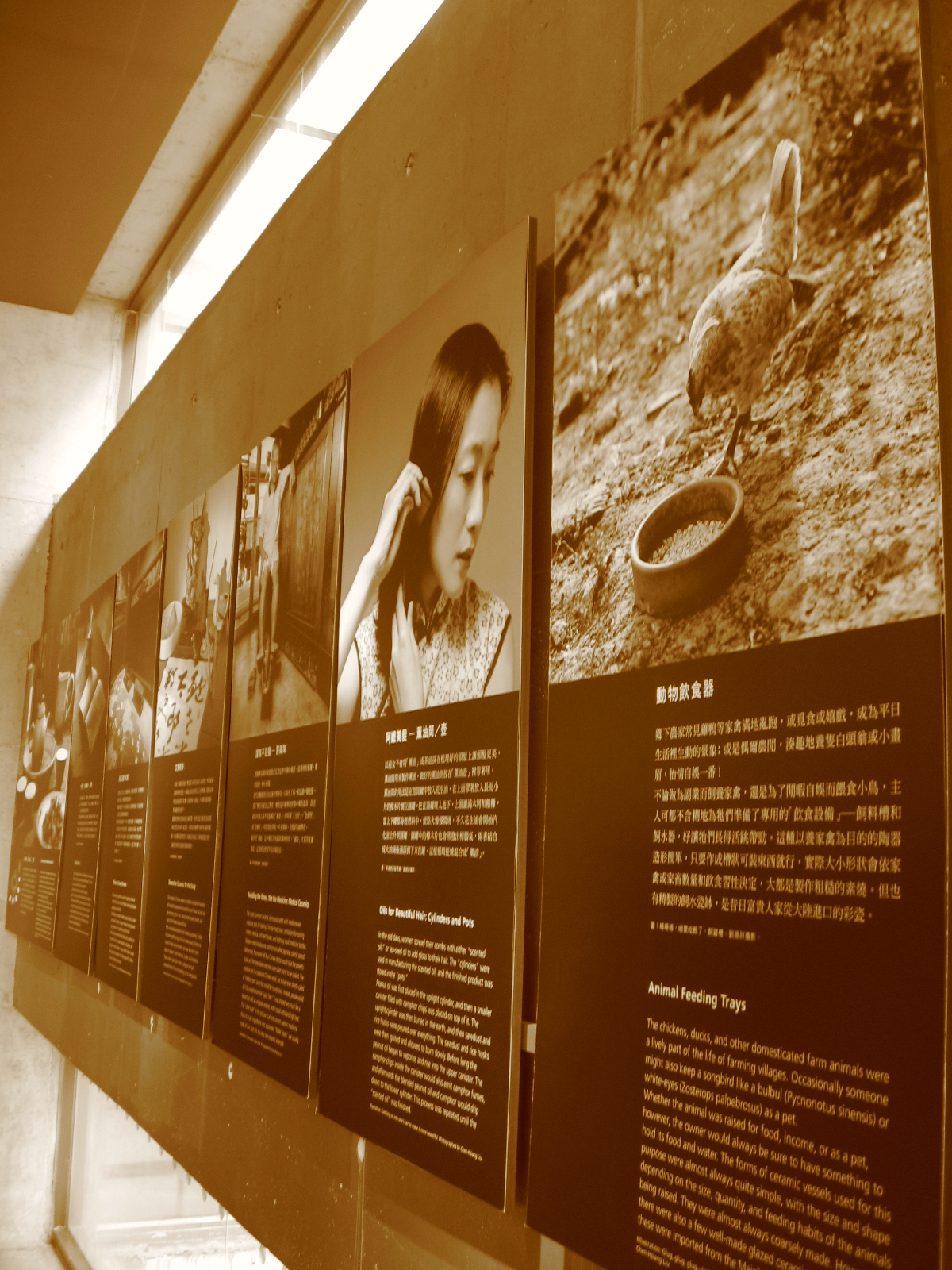This sepia-tinted photograph captures an indoor scene within a museum-like space. The image is in portrait orientation and shows a wall adorned with large vertical posters lined side-by-side. Each poster features a photograph on the upper half, accompanied by captioned text in an Asian language followed by English explanations. The foreground poster prominently displays a bird, likely a chicken or pigeon, eating from a stone bowl, with bold white text reading "Animal Feeding Trays". Below it, the English text mentions the cultural significance of animal feeding trays in farming villages, highlighting domesticated farm animals such as chickens, ducks, and occasionally songbirds like the bulbul. The next poster features a young Asian woman in a floral print dress, gazing to her left while touching her hair. Further down the line, another poster shows a man standing near a wall, although details blur into the distance due to the depth of perspective. The entire composition has a representational realism style, blending historical documentation with cultural storytelling.